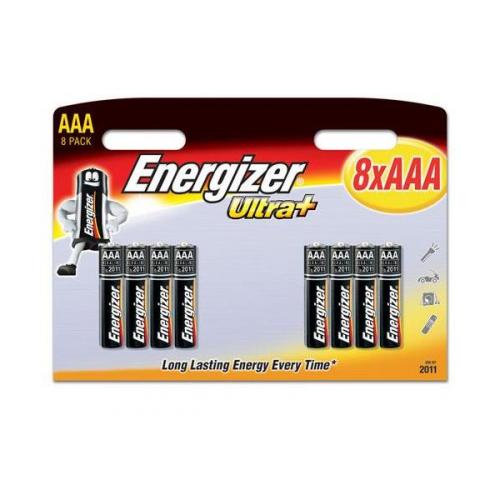The image showcases a package of Energizer Ultra Plus AAA 8-pack batteries. The packaging is neatly divided, with four batteries on the left side and four batteries on the right side, leaving an empty white space in the center. Prominently displayed at the top left is the label "AAA" in bold yellow font, with "8-pack" written just below it in a smaller size. Above the batteries, there are two oval cutouts designed for hanging the package on a retail shelf. Below these cutouts, in large, bold font, is the "Energizer Ultra Plus" branding. Adjacent to this, there is a cartoon character representing a battery, complete with a face, large muscular arms, and sneakers, albeit with one leg not visible.

Adding to the details, a bright yellow circle towards the upper section of the package highlights "8X AAA" in striking bold red font. At the bottom, a tagline reads, “Long Lasting Energy Every Time,” emphasizing the product’s reliability. The right panel of the packaging features various icons, including a flashlight and a speaker, which suggest suitable applications for the batteries. Additionally, the date "2011" is printed at the bottom right corner, indicating the production year or design iteration of the packaging.